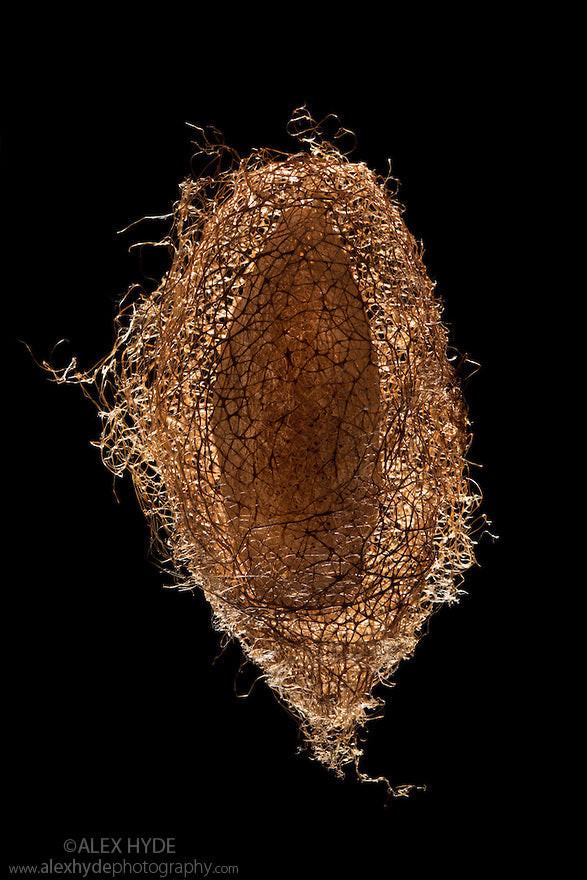The image features a wispy, abstract object crafted from thin, gold wire, intricately woven into an oval-like shape, reminiscent of dried hay suspended against a stark black background. The bottom left corner of the photograph bears a faint, light-colored font with the text "copyright Alex Hyde" followed by the URL "www.alexhydephotography.com," where "Hyde" is spelled H-Y-D-E.